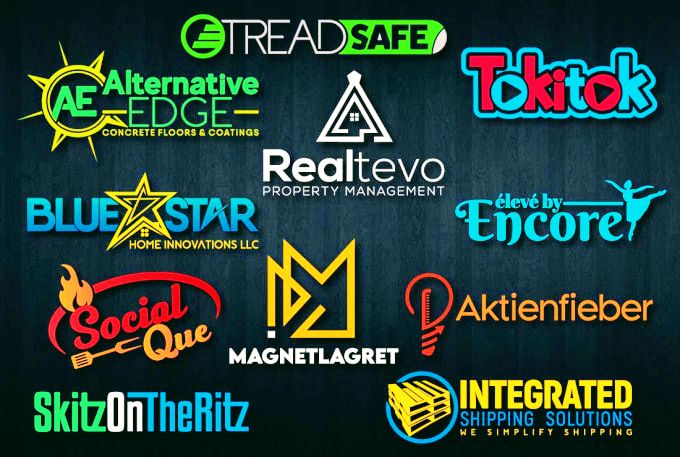The image displays a flyer or advertisement with a dark blue to black gradient background, resembling a wooden wall with varying light intensity. The brand names are positioned around the edges and some in the center, each offering different services, many related to construction. From the top left, the flyer features "Treadsafe" and "Alternative Edge Concrete Floors and Coating." In the top middle is "Real Tevo Property Management," and at the top right is "Talky Talk." Moving down the right side, there's "Elevate by Encore," followed by "Acti and Fiber," and at the bottom right, "Integrated Shipping Solutions - We Simplify Shipping." In the center bottom, "Magnet Lagrit" is highlighted. On the middle left, there's "Blue Star Home Innovations LLC," with "Social Q" below, and at the bottom left, "Skits on the Ritz." The brands cover a variety of services ranging from property management and construction to social services and shipping.